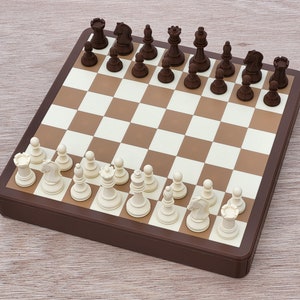The image showcases a pristine, high-quality chess set rendered in a detailed, slightly tilted aerial view. The chessboard, slightly raised about an inch or two, features a dark brown border with alternating off-white and medium brown squares. The pieces—typical chess pieces in cream and dark brown—are meticulously aligned in their starting positions with the cream pieces closer to the viewer and the dark brown pieces farther away. The board is tilted about 45 degrees to the right, resulting in the upper right and lower left corners being just cut off by the edge of the image. The entire setup rests on a light-colored wood grain surface, likely a white oak, contributing to a bright and vibrant overall appearance. The absence of other elements in the background and the perfect alignment of pieces suggest the image might be a 3D rendering or heavily photoshopped. The chess set, with its orderly arrangement and high-end finish, presents a clean, professional aesthetic.